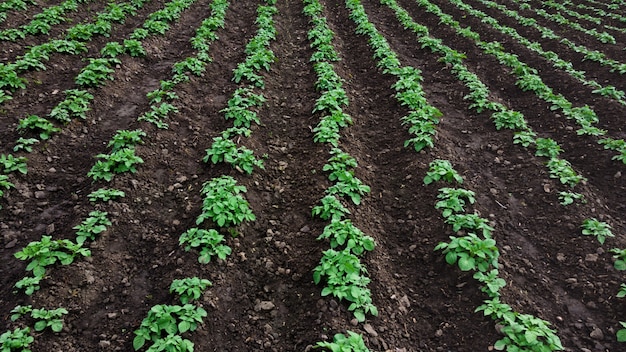The image depicts a meticulously tended farm garden, showcasing approximately 10 to 15 well-organized, straight rows of lush, bright green potato plants. The potato plants, each about two to three inches tall, are robust and leafy, with some larger and some smaller plants visible. The rows, appearing slightly elevated, form distinct raised beds with narrow channels of dark, almost black soil in between. The soil, seemingly just watered, contrasts sharply with the lighter-colored rocks and clumps of dirt scattered throughout the channels. Footprints in the mud indicate recent human activity, suggesting attentive care of the healthy potato plants. The photograph, taken at a slight aerial angle, captures the rows of plants extending out toward the top of the frame, emphasizing the orderly and thriving nature of this productive garden.